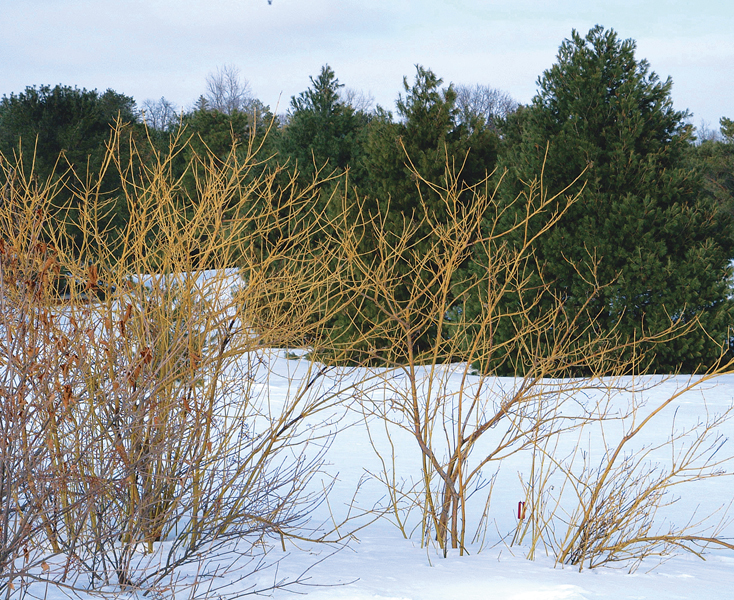This photograph captures an outdoor winter scene dominated by a pristine blanket of white snow covering the ground, with various types of trees scattered across the landscape. The sky above is overcast, featuring light gray clouds that cast a subdued, diffuse light over the scene. Centrally placed in the foreground are several tan-colored, leafless bushes or small, bushy trees, comprised of hundreds of thin branches, some extending up to six or eight feet tall. These branches become denser towards the left side of the image and more sparse towards the right. 

In the background, rows of deep green pine trees stretch as far as the eye can see, interspersed with a few taller, deciduous trees stripped bare of their leaves for the winter. The stark contrast between the vibrant green of the pine needles and the light brown branches in the forefront enhances the scene's depth and complexity. The snow appears undisturbed, devoid of any footprints or tracks, laying flat and clean. High above in the light blue sky, partially obscured by clouds, a small black dot can be seen—potentially a bird in flight, adding a subtle dynamic element to the tranquil winter landscape.